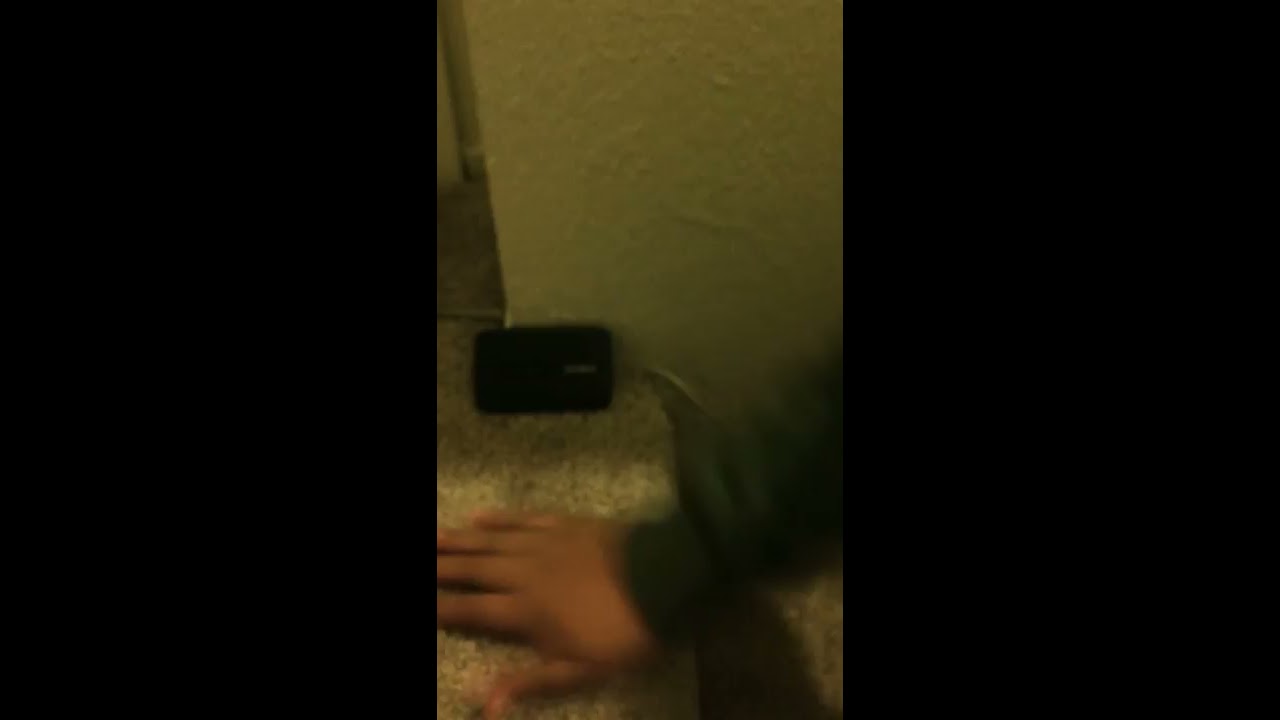The image is a square picture, predominantly dark, featuring a man's right hand placed on a table or counter. The overall setting is dimly lit, creating a somewhat blurry and distorted effect. The man's hand, which is of a darker skin complexion, extends from a long-sleeve shirt that appears to be a dark color, possibly green. The background consists of a rough, stucco-like white wall. On the table near the hand, there is a small, three-dimensional black box with a bit of white marking, possibly a logo or scuff, in the bottom right corner. The left side and the back right side of the image are particularly dark, emphasizing the central elements of the hand and the box. Additionally, there is a slight view of a floor angle to the left of the wall, contributing to the image's overall dark and blurry ambiance.